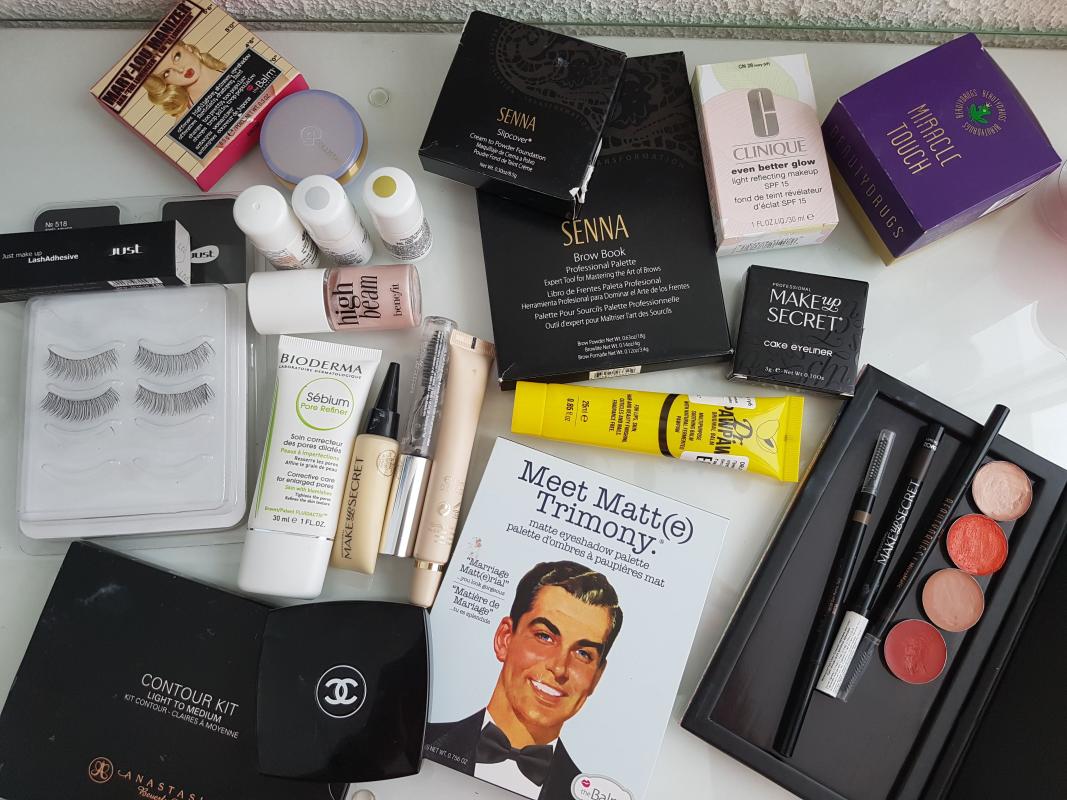A meticulously arranged glass vanity, with a pristine white surface beneath the glass, showcases a diverse collection of makeup products. Let's start our tour in the lower left-hand corner where a black bag labeled "Contour Kit Light to Medium" is stationed. Resting on top of this bag is a sleek makeup compact adorned with two interlocking C's, likely the emblem of Chanel.

Moving clockwise, directly above the bag, we spot a case designed to hold four sets of fake eyelashes, though two sets have already been used. Adjacent to this is a bottle of Bioderma serum, complemented by three miniature tubes, possibly mascaras, each featuring a small brush attachment. Just above this group is a bottle marked "High Beam" surrounded by a collection of short, stubby bottles with gray and greenish tints on their lids, presumably nail polishes.

Continuing to the topmost area, we come across a box featuring an illustration of a retro-styled girl with the inscription "Mary Lou." Nearby, there's another compact and a larger box identified as "Senna Brow Book." Moving rightwards, a box from Clinique labeled "Even Better Glow" sits next to a purplish box branded with "Miracle Touch." Slightly lower, an eyeliner marked "Makeup Secret" is accompanied by a yellow tube bearing the name "Dr. Paw Paw."

Further to the right, a set of eyebrow pencils resides in a small black box alongside four pots of blush in varying shades. Centrally positioned towards the bottom of the display, a retro-themed card labeled "Meet Matt Tremoney" alongside "Matt Eyeshadow Palette" adds a charming vintage flair, rounding out this meticulously organized and impressive assortment of beauty essentials.